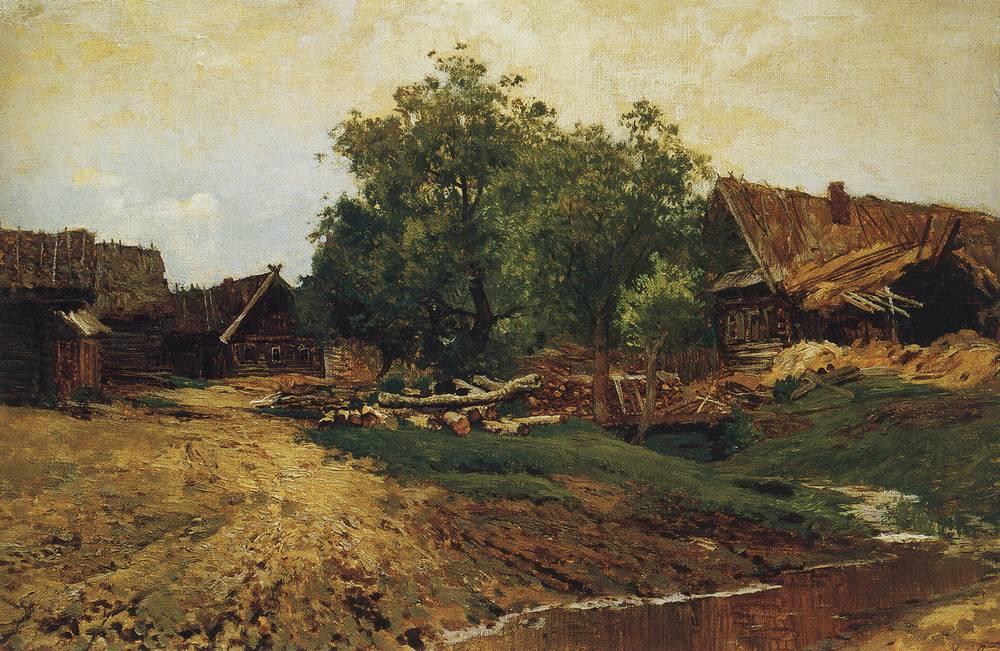The watercolor painting captures a serene daytime scene of a rural countryside. The sky is a mix of blue and white with hints of brown, streaked with soft clouds. Central to the image are lush, green, leafy deciduous trees, interspersed with a few felled, log-like branches scattered on the ground. The right side of the painting features an old, rustic cabin with a wooden roof and chimney, surrounded by straw debris, suggesting its worn, dilapidated state. Adjacent to the cabin, a small brook flows, bordered by the bridge laden with logs that connects the property to a dirt road extending to the foreground. This road leads to the left side of the painting, where another cluster of old wooden houses and what seems to be a barn are situated. Together, these elements convey a nostalgic, pastoral setting, with a dirt road linking the scattered buildings amidst the gentle, natural landscape.